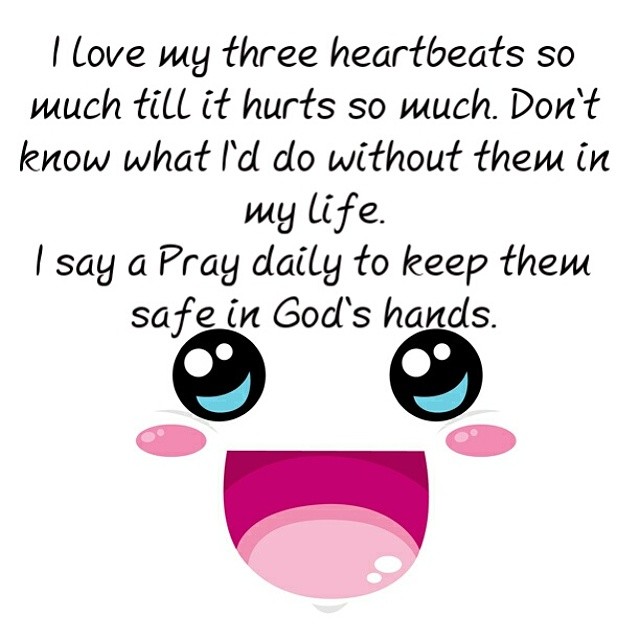The image is a computer-generated postcard featuring a cartoon-like smiley face at the bottom with asymmetrical eyes—one big and one small—with black pupils accented in white and blue. The face has rosy cheeks, a blue mouth, and a visible pink tongue, giving it a cute and playful appearance. Highlighted above the smiley face in cursive black text, the message reads: "I love my three heartbeats so much till it hurts so much. Don't know what I'd do without them in my life. I say a prayer daily to keep them safe in God's hands." The background is plain white, accentuating the vibrant design elements, including the shades of bright and darker pinks that appear to form additional facial features below the smiley face, adding to its expressive look. A small gray element is also visible under the design. The overall aesthetic is a blend of whimsy and heartfelt sentimentality, typical of inspirational social media posts.